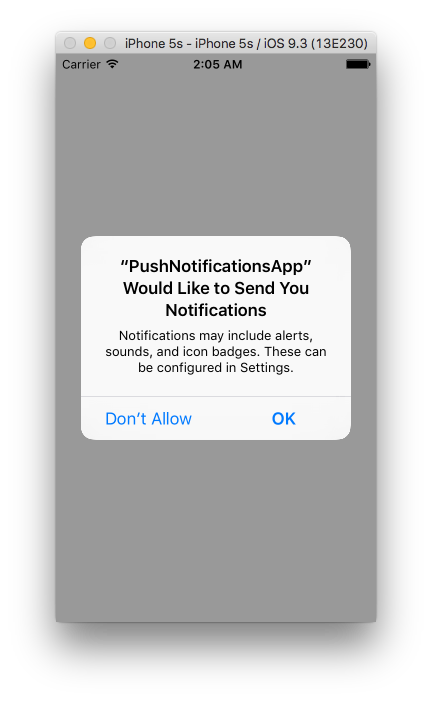A pop-up notification appears on an Apple iPhone 5s running iOS 9.3 at 2:05 a.m. The notification, labeled "Push Notifications App," requests permission to send notifications. The message states: "Push Notifications App would like to send you notifications. Notifications may include alerts, sounds, and icon badges. These can be configured in Settings." Below this message, two options are provided: "OK" and "Don't Allow." The background behind the pop-up is a dark gray screen.